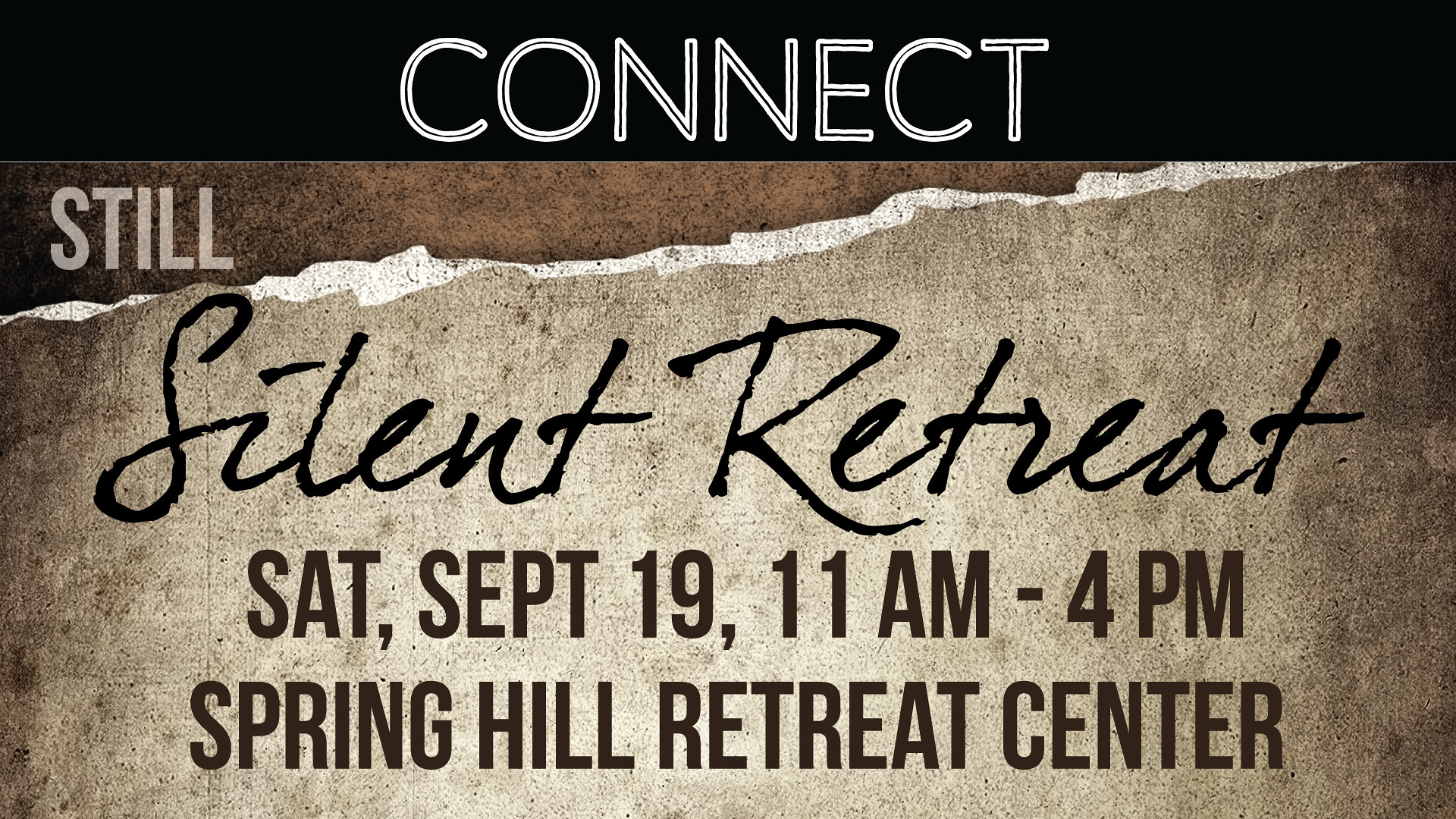The image depicts an intricately designed advertisement for an event. At the top of the poster, in a white bold font, is the word "CONNECT" set against a solid black background strip that spans the width of the sign and takes up about an eighth of its height. Below this, there appears a torn piece of paper effect with rugged edges revealed in dark brown. Set against this, in a beige font, is the word "STILL."

Centrally positioned on this textured brown segment in a dark brown script font are the words "Silent Retreat," with only the 'S' and 'R' capitalized, emphasizing the casual, handwritten feel. Beneath this in all capital letters are the event details: "SATURDAY, SEPTEMBER 19TH, 11 A.M. TO 4 P.M., SPRING HILL RETREAT CENTER," etched in the same dark brown, providing a stark yet cohesive contrast.

The lower portion of the image is lighter, featuring shades of tan and giving an impression of a stone or cement background. The overall color palette consists of browns, beiges, whites, and specks of black, contributing to a rustic, serene aesthetic that aligns with the retreat's theme.